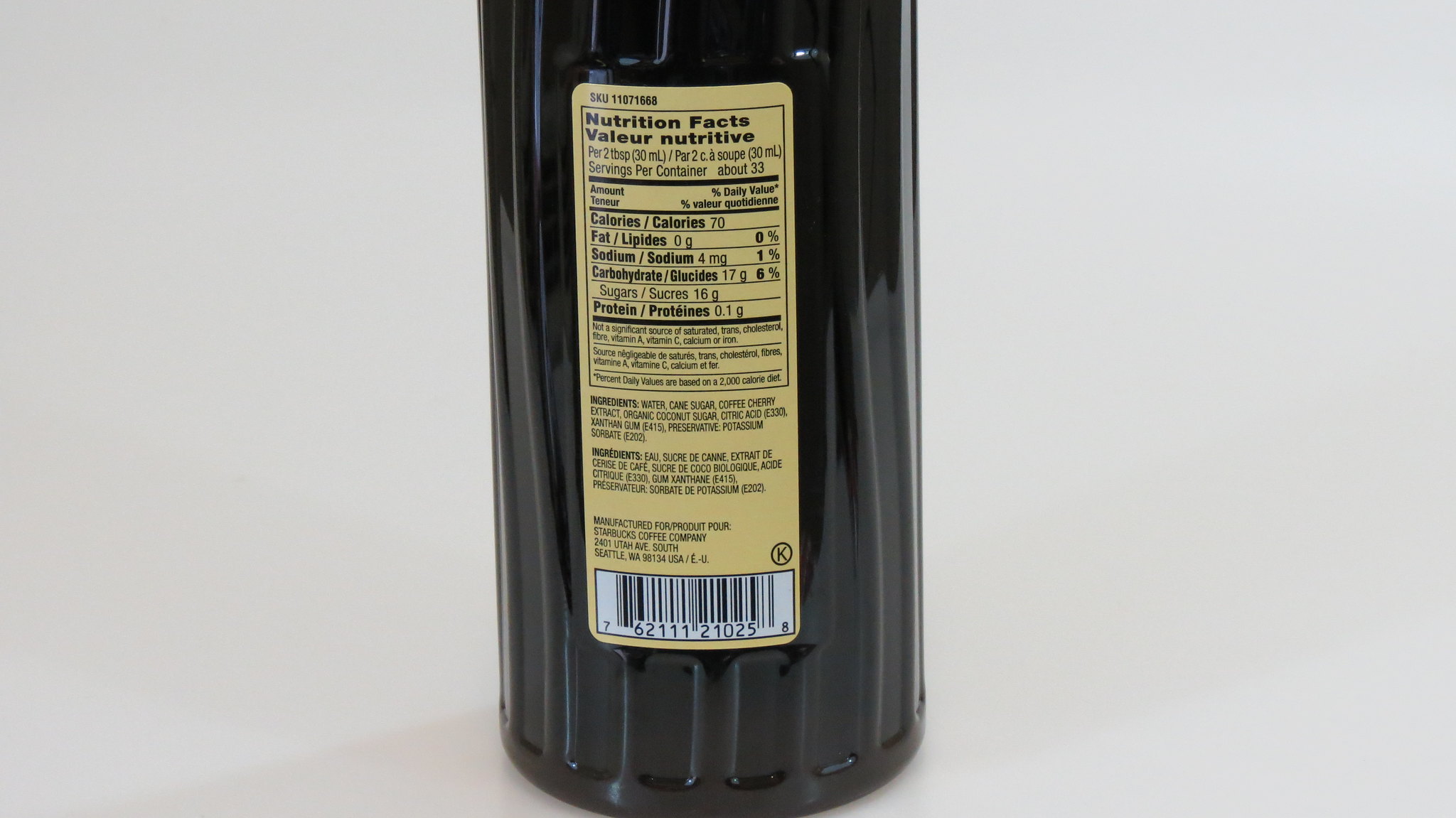The image depicts a textured bottle, filled with a dark liquid, positioned on a pristine white surface with a matching white background. The back of the bottle features a prominent yellow label with black text. The label details nutritional information, including "Nutrition Facts" and "Value Nutrient," highlighting that the liquid contains 70 calories, 0 grams of fat, and lists the amounts of sodium, carbohydrates, and protein. At the bottom of the label, a barcode is visible, along with a sequence of numbers beneath it.